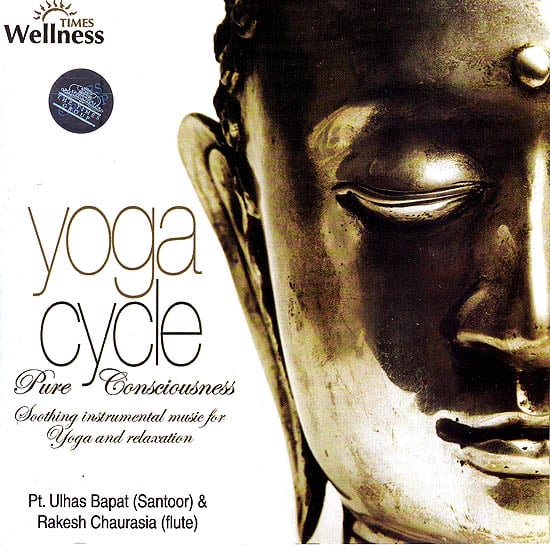The image appears to be a cover, possibly for a CD, designed for a soothing and meditative theme. On the top left corner, the text "Times Wellness" is prominently displayed, accompanied by a drawing of a sun above it. Below this, a small circle, grey or black in color, bears the text "The Times Group" along with a crown.

The main title "yoga psycho" is written in large, bold, lowercase letters. Beneath this, in elegant cursive, is the subtitle "Pure Consciousness Soothing Instrumental Music for Yoga and Relaxation." 

On the bottom left corner, the musicians are credited: "PT Ulhas Bapat (Santoor) and Rakesh Chaurasia (Flute)." 

Dominating the right half of the image is a golden sculpture of a person's head, depicted from the forehead to the chin and only showing one side of the face. This half-face includes one eye (which is closed), half of a nose, and a mouth. Notably, a gold dot or mark is placed on the forehead. The statue, with its elongated earlobes and serene expression, might represent an Indian deity.